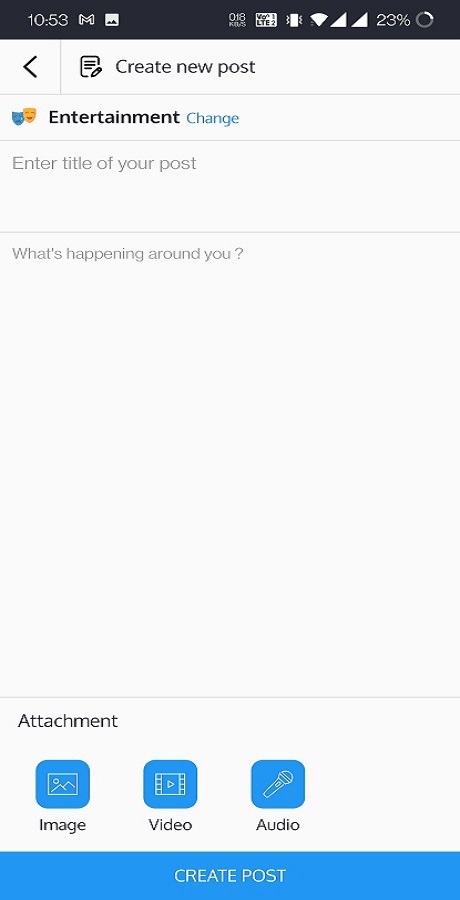This image captures a smartphone screen displaying a social media platform's interface. 

At the top, a thin black banner displays the time "10:53 AM" in white text. To the right of the time, a series of icons are present: a white square with a red outline featuring a mountain-like design with two black peaks, followed by "018" and another white square with the text "V01LTE2" inside. Next, a vertical rectangle with zigzag edges is seen, accompanied by a Wi-Fi symbol and two cell signal bars. The battery icon shows a 23% charge with a partially filled white circle extending from the 12 to 2 o'clock position.

Below this top banner, an arrow pointing left is visible, followed by an icon representing a piece of paper with a pencil at the bottom alongside the text "Create new post."

Further down, a theater mask icon displays a blue sad and yellow happy face, labeled "Entertainment Change." "Entertainment" is in bold with a capital "E," while "Change" appears in blue text with a capital "C."

Directly below, a text field prompts the user to "Enter title of your post," followed by a section asking, "What's happening around you?" with a question mark.

At the bottom of the screen, there are options for attaching an image, video, or audio file. A blue banner at the bottom reads "Create Post."